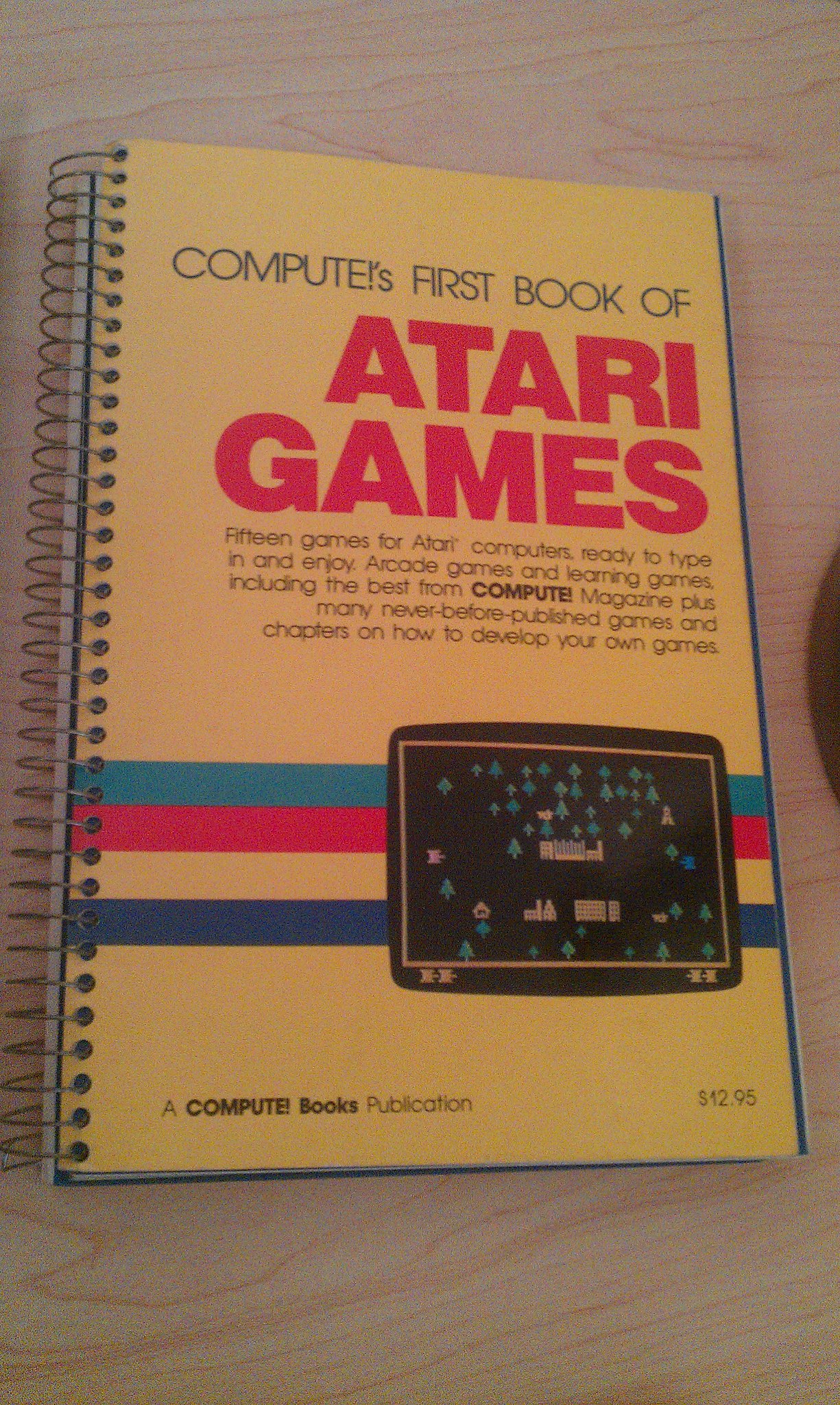In the image, a spiral bound book titled "Compute's First Book of Atari Games" rests on a table showcasing a light white surface with brown wood grain patterns. The yellow cover of the book prominently features black text stating "Compute's first book of" followed by bold red text spelling "Atari games." Beneath this title, additional details in black text declare, "15 games for Atari computers ready to type in and enjoy. Arcade games and learning games, including the best from Compute magazine, plus many never before published games and chapters on how to develop your own games." The cover also displays four horizontal stripes in blue, pink, yellow, and blue, just above an image of an Atari screen depicting trees and buildings. In smaller black text at the bottom left, it reads "a Compute Books publication," while the bottom right corner shows a price of "$12.95." The spiral wire binding on the left side of the book and the overall grainy quality of the image add a vintage feel to the scene.